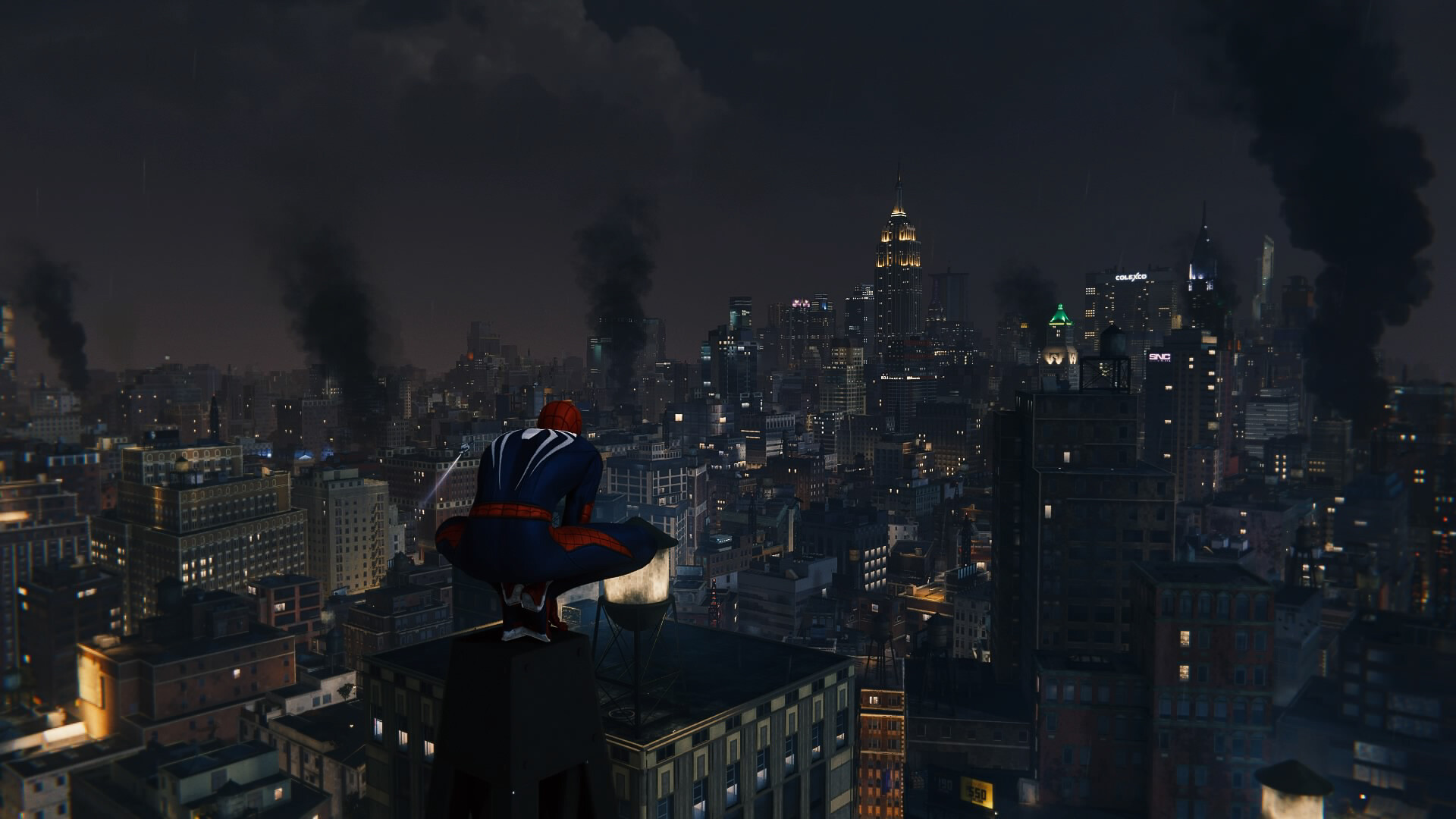The image depicts a cityscape at nighttime, rendered with apparent AI or computer-generated artistry. Dominating the scene is Spider-Man, who is perched atop a smokestack or a spire. He is crouched down, balanced on the balls of his feet with his knees bent and spread wide, bending forward as he gazes down at the expanse below. His iconic red and blue suit is visible, with a predominantly dark blue color, accented by a red mask, a red belt, and possibly some red detailing on the pants. 

The city below is bathed in dark, muted shades of gray and black, creating a somber atmosphere. The sky is a deep gray, with a faintly visible cloud adding to the moodiness of the scene. From five distinct locations, black smoke billows upwards, signifying industrial activity or perhaps turmoil.

The city's architecture is a tapestry of tall, narrow buildings, most topped with flat roofs. Though predominantly lit by white lights, there are sporadic bursts of color: light blue lights scattered here and there, a singular light green source positioned high up, and a few yellow lights closer to the ground. The overall effect is a sprawling, almost oppressive urban landscape punctuated by pockets of luminosity.